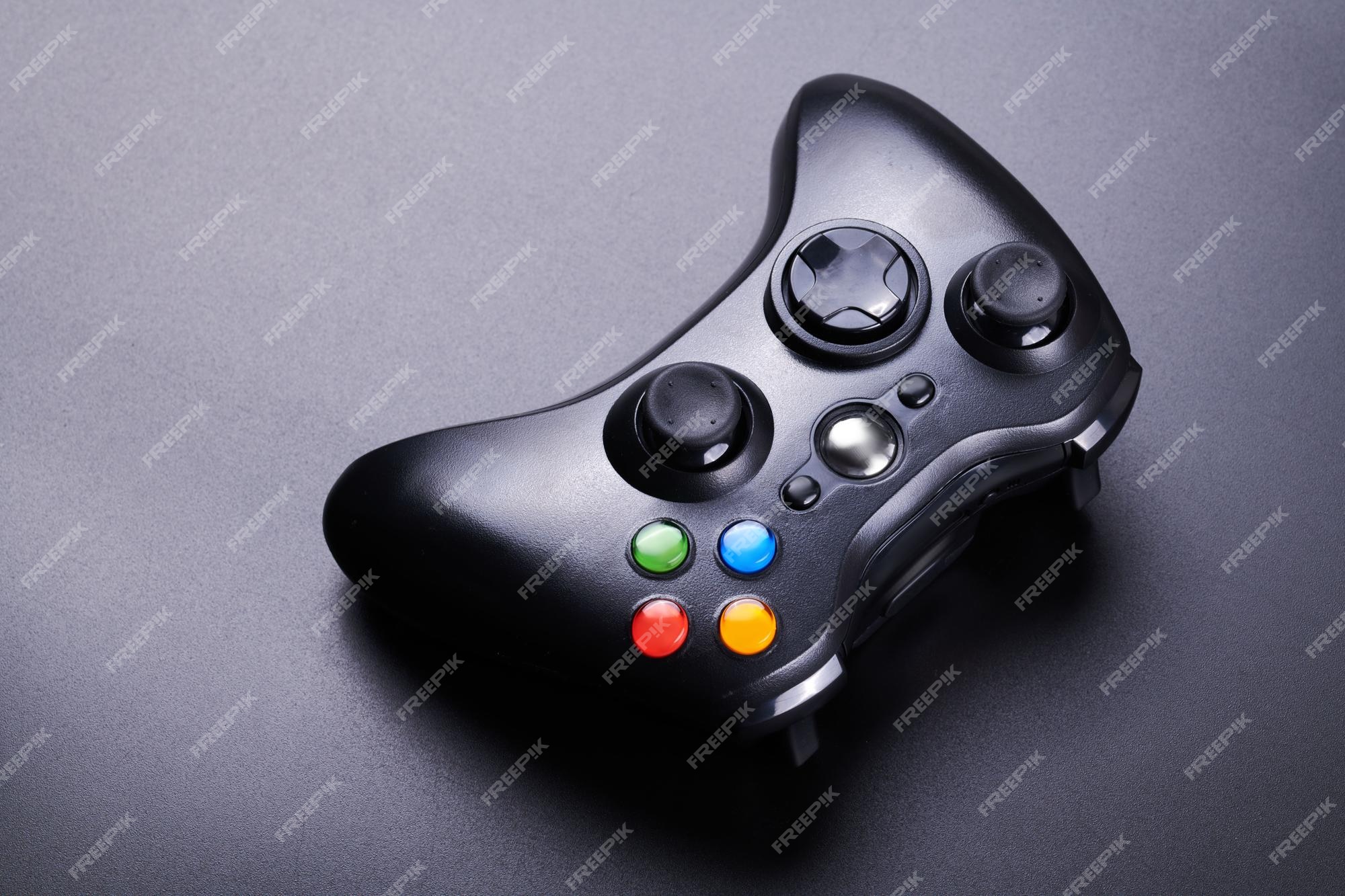This photograph features a generic black video game controller reminiscent of those used for Xbox or possibly PlayStation, although it lacks specific branding. The background is a dark gray overlaid with diagonal "FREE PICK" watermarks in all caps, with the 'I' resembling an exclamation point. The controller dominates the image, though it is not perfectly centered and is placed at a right angle. The device is equipped with dual black joysticks, a D-pad, and four colored buttons: red, green, blue, and yellow. Additionally, there are three central buttons; two small ones and a larger silver one. The glossy black controller, which takes up most of the frame, appears to be wireless, with no cord attached.